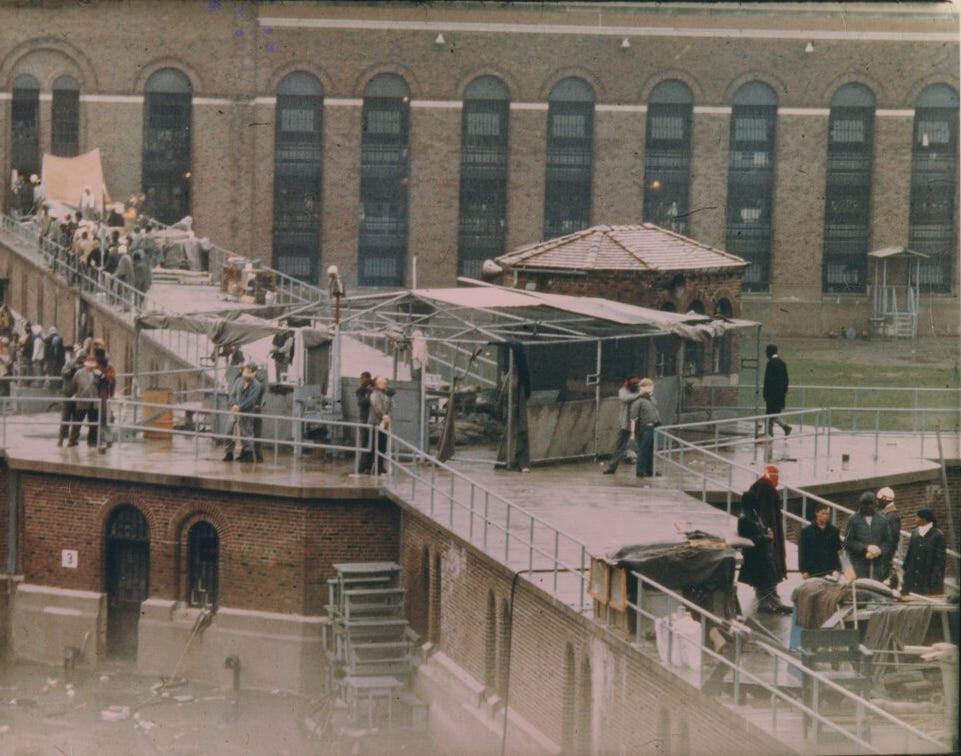The image captures an outdoor urban scene dominated by a large brown brick building featuring tall, arched windows. In the foreground, there is a walkway on top of a smaller structure, surrounded by silver-colored railings that extend into various directions from a central point—one path continues straight, while two others veer off to the left and right. The walkway starts from the bottom right of the image, where a ladder is propped against a brick wall that transitions to light gray concrete below. Scattered along the walkway are a few chairs and miscellaneous items, potentially obstructing the path. The scene is bustling with numerous people, both on the upper walkway and at the ground level. The lower part of the building features an arched doorway and a similarly arched window. The environment gives a sense of either a movie set or a prison, suggested by the building's imposing structure and the mix of people occupying both levels. In the background, the taller main building looms with its numerous arched windows, contributing to an air of organized chaos in this expansive, multifaceted scene.